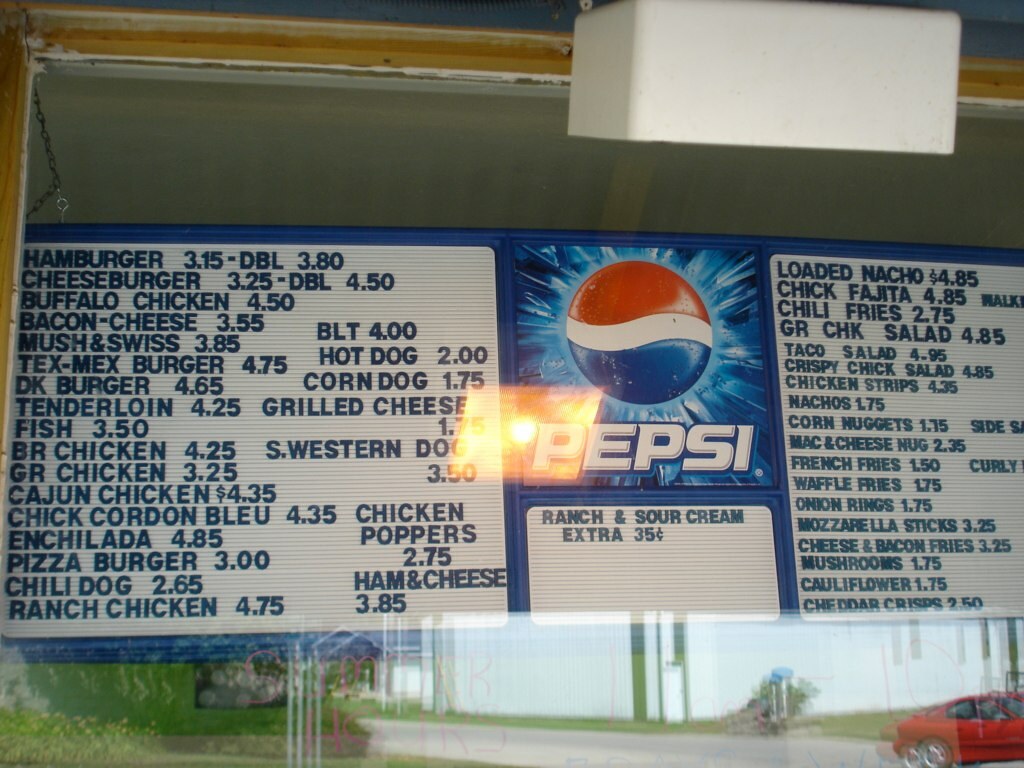In the photograph, we see the outside of a brown window frame with reflections that add depth and context to the image. A blue menu sign, prominently featuring the Pepsi logo at the center, is visible through the window. The menu is divided into three distinct sections. The left section lists a variety of food items including hamburgers, cheeseburgers, buffalo chicken, bacon cheese, mushrooms and Swiss burgers, Tex-Mex burgers, DK burgers, tenderloin, fish, chicken BLT, hot dogs, corn dogs, and grilled cheese among other offerings. The central section highlights that ranch and sour cream are available for an additional cost of 35 cents. The right section displays options like loaded tacos, nachos, chicken fajitas, chili fries, GR chicken salad, waffle fries, and various sides.

Reflective surfaces in the window show a red car at the bottom right corner of the photo, and at the bottom left, there are images of a white building, a street with mailboxes, and some flowers and bushes. A white box, likely a light fixture, is attached to the front of the window frame, adding a practical element to the restaurant's exterior. This well-detailed scene captures the essence of a local eatery, giving a glimpse of its offerings and surroundings.